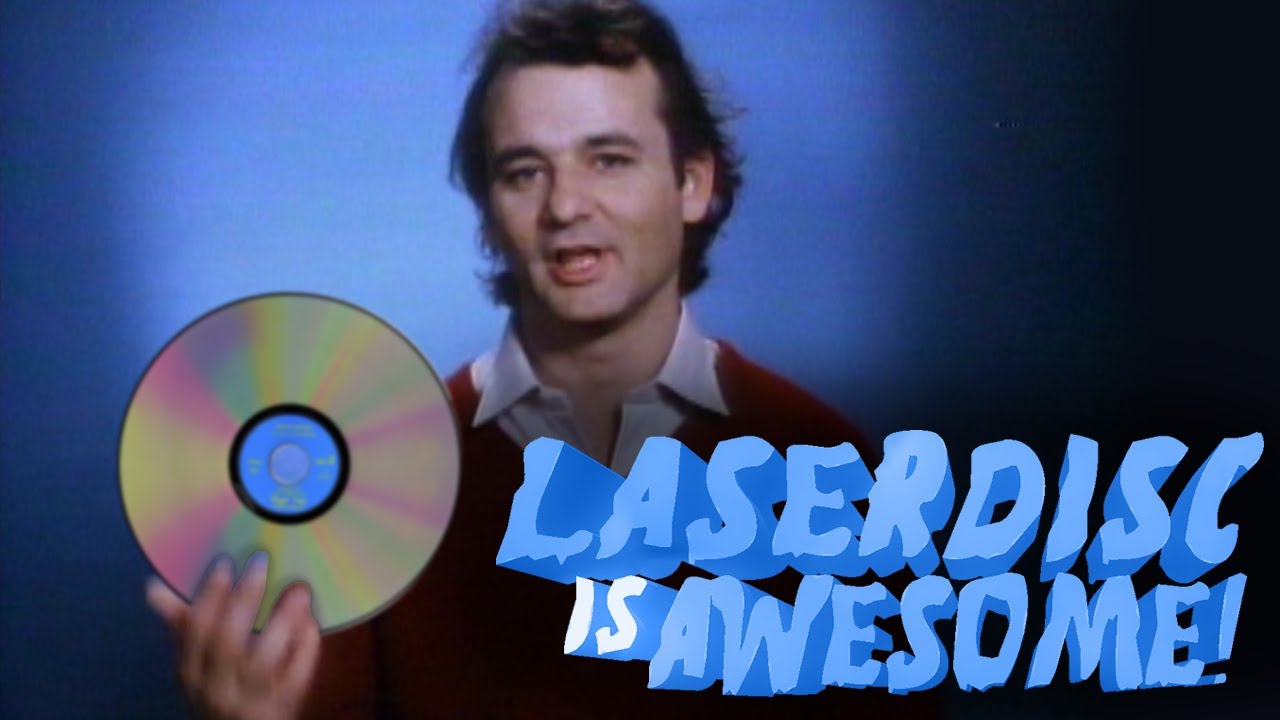The image is a rectangular, color advertisement featuring a younger Bill Murray against a gradient background that transitions from light blue on the left to dark blue on the right. Murray, sporting brown hair and an open-mouthed expression as if speaking, is seen from the shoulders up. He is dressed in a red sweater layered over a white collared shirt. In his right hand, he holds an unrealistically large, multi-colored disc, presumably photoshopped in. The bottom right corner displays the words "LASER DISC IS AWESOME!" with "LASER DISC" and "AWESOME" in light blue, three-dimensional capital letters and "IS" in white text, accompanied by an exclamation point. The setting is well-lit, emphasizing the clarity and vibrancy of the image.